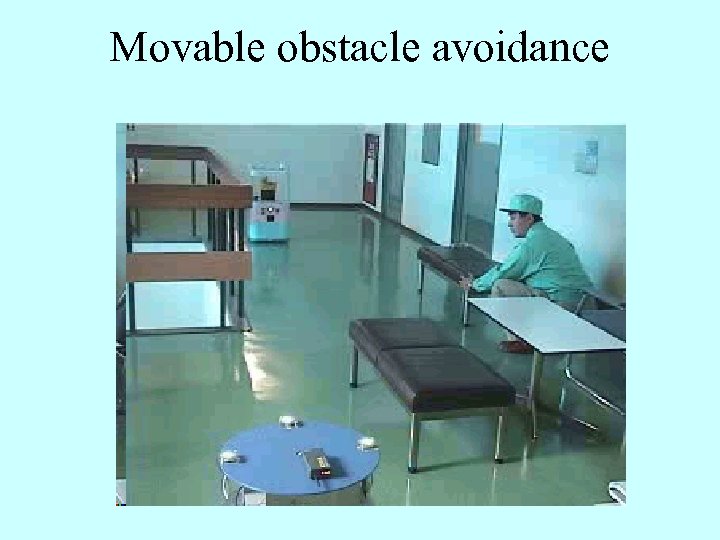The image appears to be an instructional scene set in a clinical-looking, multi-floor building such as a hospital or office. The setting resembles a large waiting room with tiled, shiny brown or gray floors. The walls are painted white, and there are two brown doors with windows at the top. On the left side of the image, there's a railing made of brown and black materials, indicating the room is on an upper floor from which you can look down.

In the foreground, there is a small round table with a blue tabletop and an unspecified object on it. Central to the image is a two-seat bench with brown cushions and silver legs, placed in front of a rectangular white table. A man is seated on the right side of the room, against a white wall, wearing a green cap, a long-sleeve green shirt, khaki pants, and brown shoes. It appears he is moving one of the seats. The image is bordered by a light blue background, and at the top, black text reads, "movable obstacle avoidance." The colors in the room include various shades of brown, gray, white, light blue, black, and turquoise, giving it a somewhat educational and clinical ambiance.